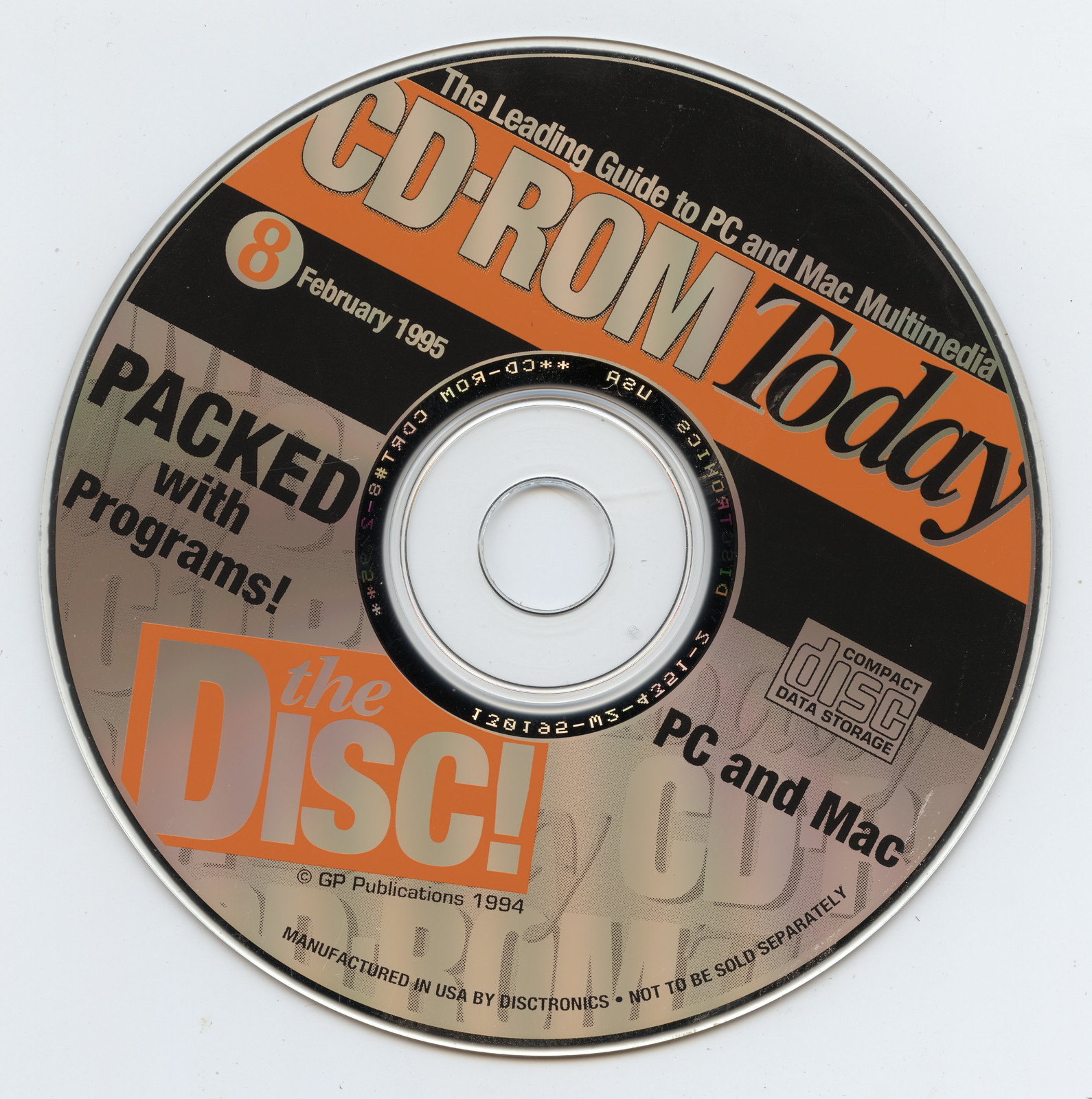The image features a single black and orange CD prominently centered against a stark white background. Positioned diagonally with a slight tilt to the right, the CD's upper section displays the white text "The Leading Guide to PC and Mac Multimedia." Below, an orange strip boldly states "CD-ROM Today" in white and black text. The middle part of the CD includes a black strip with the date "8 February, 1995" in orange text. The lower half is predominantly gray, bearing the text "Packed with Programs, PC and Mac Compact Disc Data Storage," with "The Disc" highlighted in an orange box with white text beside the GP Publications 1994 mark. Encircling the central circular cutout are additional details, including "Manufactured in USA by Discotronics" and a note, "Not to be sold separately." The CD rests slightly off-center, giving the overall image a balanced yet dynamic feel.